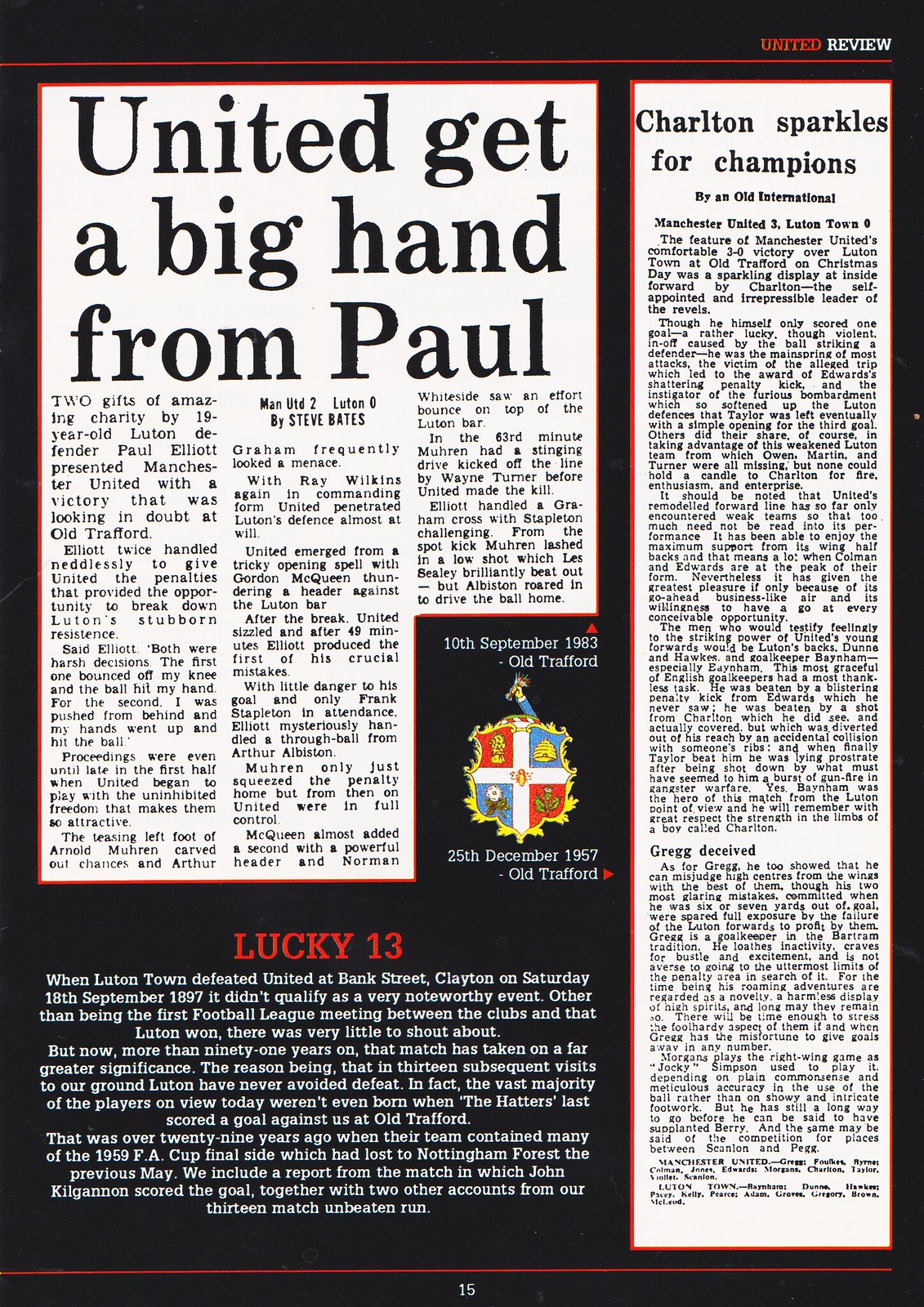The image is a page from a magazine, featuring two distinct news articles. The left article, formatted with black text on a white background, prominently headlines: "United get a big hand from Paul." It details how 19-year-old Luton defender Paul Elliott's two inadvertent handballs gifted Manchester United a victory that seemed uncertain at Old Trafford. Elliott explained that the first incident occurred when the ball deflected off his knee onto his hand, while the second happened as he was pushed from behind, causing his hands to hit the ball. Until late in the first half, the game was evenly matched, but United eventually capitalized on these penalties to overcome London's resilient defense. The article captures the tension and eventual breakthrough, noting United's expressive style of play. Additionally, a logo located towards the center of the page marks the dates "10th September 1983" and "December 25th, 1957," both referencing Old Trafford, further situating the historical context of the events discussed.